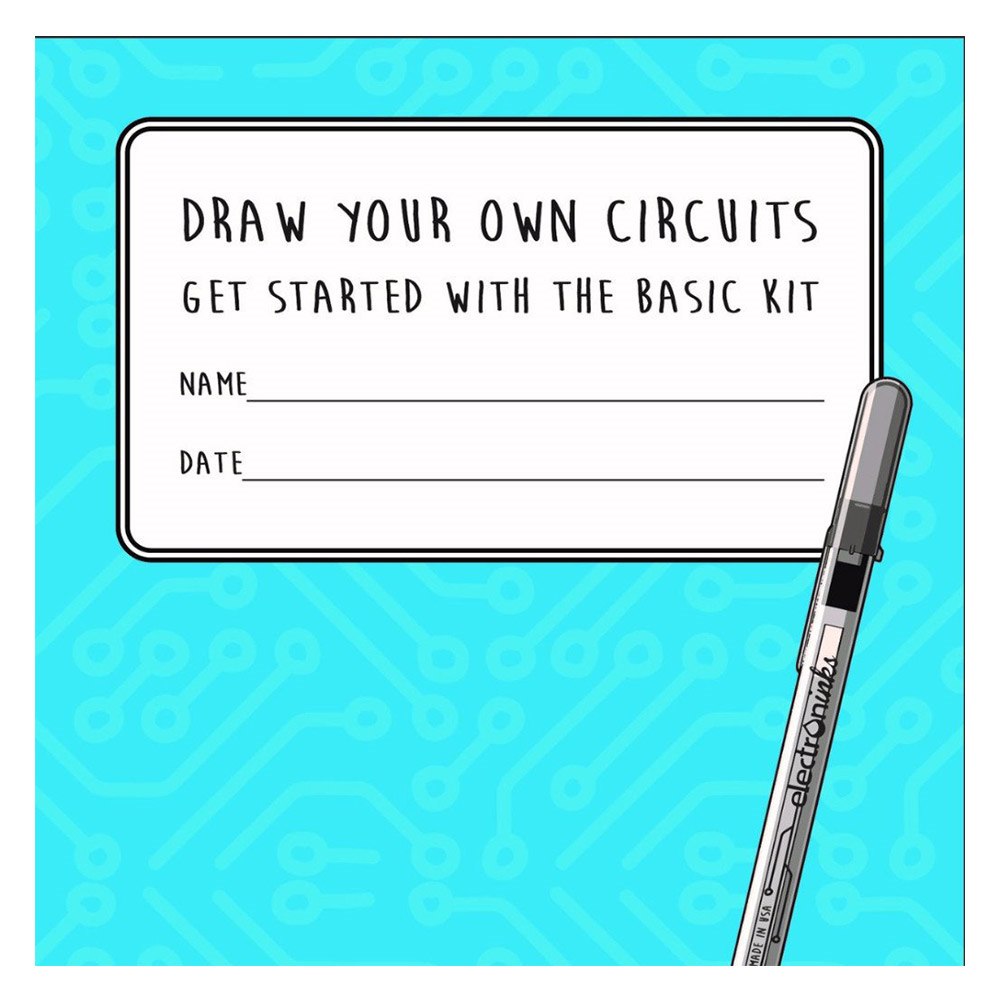The image features a digitally created scene with a blue background adorned with a circuitry pattern in a lighter shade of blue. Centrally positioned, slightly above the midpoint, is a white rectangle with a black outline resembling a piece of notebook paper, containing the handwritten text "Draw your own circuits, get started with the basic kit." Beneath this text are two lines labeled "Name" and "Date." In the bottom right corner of the image lies a silver pen with a black cap, featuring the text "Made in USA" and "Electronics" in a stylized font. The overall design evokes a scholastic or educational theme.